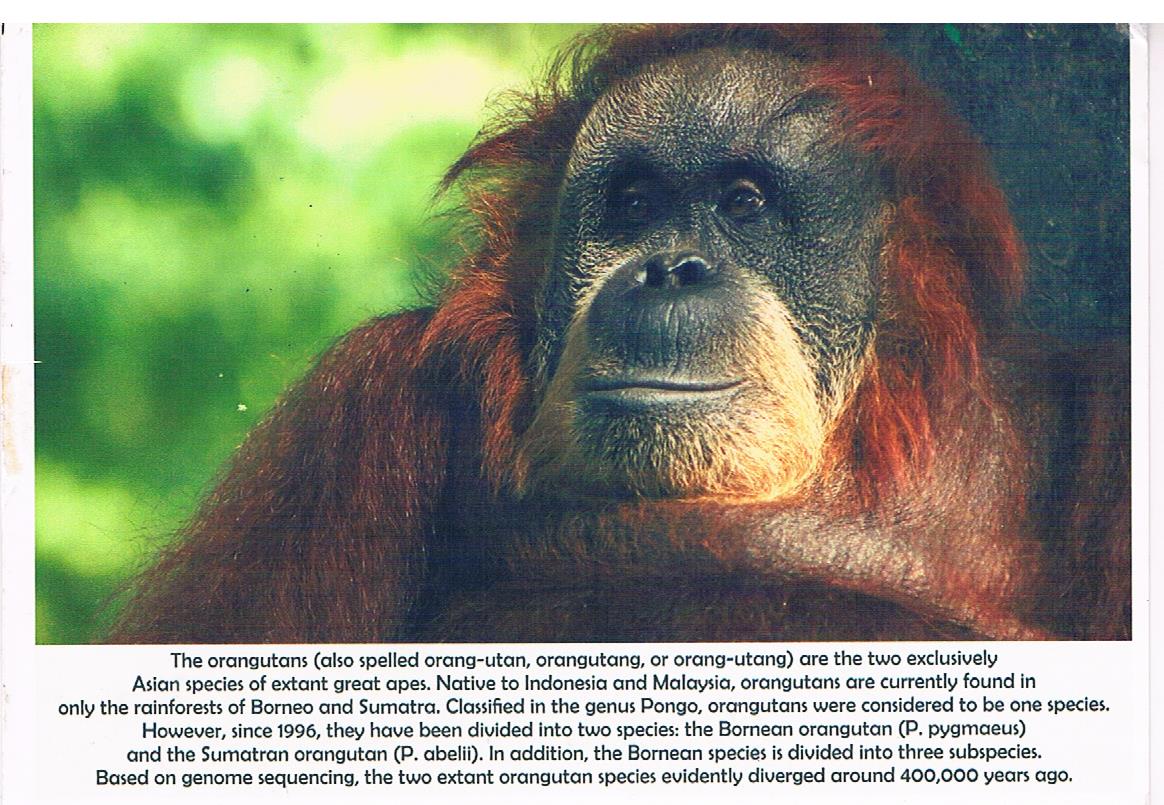The image depicts a close-up of an orangutan scanned from a magazine article, possibly from a publication like National Geographic. The orangutan, with its distinctive reddish-brown fur and blackish-brown skin, is situated outdoors in its natural habitat. Its eyes are open, looking slightly to the side, giving it a somewhat startled expression. The background features a blurred, marbleized green color with dark gray in the corners, focusing the viewer's attention on the orangutan. Accompanying the image is a detailed paragraph explaining that orangutans—also spelled "orang-utan"—are two exclusively Asian species of great apes found in the rainforests of Borneo and Sumatra. Classified in the genus Pongo, it details their distinction into the Bornean orangutan (P. pygmaeus) and the Sumatran orangutan (P. abelii), highlighting their evolutionary divergence around 400,000 years ago. The text is in black, providing in-depth information about these critically endangered apes.